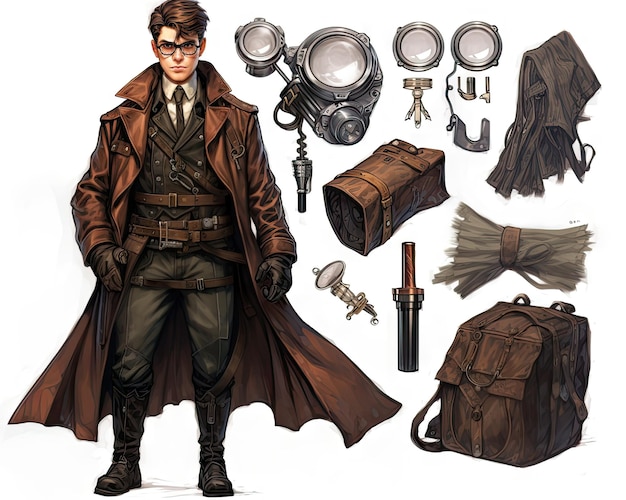The image is a detailed character concept art showcasing a young man, approximately in his early twenties, standing on the left side. He has short brown hair and wears glasses. His attire is a blend of military and old-fashioned style, featuring a dark brown or possibly dark gray suit with a white shirt and a dark gray tie underneath a long, unbuttoned brown trench coat. The coat, which may be leather, extends to the back of his legs and has a wide collar. His outfit is accentuated by numerous belts around the waist and a strap that goes diagonally across his chest. He completes his look with dark brown or black fatigue pants, high boots that reach nearly to his knees, and dark brown gloves.

On the right side of the image, an array of gear is displayed. This includes various ocular devices like eyepieces or monocles, a brown bag with leather straps, a cylindrical tube with a stick, and multiple backpacks. There's also a light gray clothing item tied with a brown band. This collection of items suggests that the character is equipped for espionage or spy-related missions.